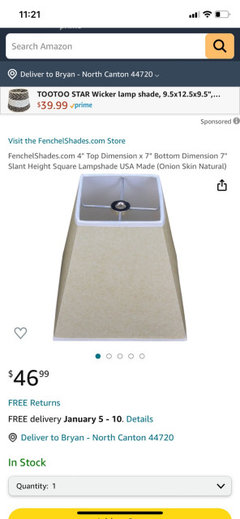**Image Description: Detailed Screenshot of an Amazon Purchase Interface**

The screenshot is taken from a cellphone on the Amazon website, captured at the top left with a timestamp "11:21" and signal strength at 3 out of 4 bars. The Wi-Fi indicator is fully lit, indicating an active connection, and the battery icon shows a partial charge.

Central to the screen is the Amazon search bar, followed by the delivery location indicated as "Delivered to Brian via YAN-NorthCanton44720." Below that, there is a promotional banner advertising a lampshade with dimensions 9.5 x 12.5 x 9.5 inches, priced at $39.99, featuring the Prime logo, and accompanied by four small navigation dots for banner browsing.

The main section of the screenshot displays an item entitled "Visit the FenchelShades.com Store". The product featured is a FenchelShades.com square lampshade with a 4-inch top dimension, 7-inch bottom dimension, and a 7-inch slant height. It is noted as "USA Made" and showcases a "Natural" finish. The image of the lampshade reveals a beige shade with white bandings, angular in structure, wider at the bottom, sloping to a narrower top. There are five dots below the image, suggesting additional product images, with the first dot highlighted in dark blue.

The product is priced at $46.99 with benefits like free returns and free delivery estimated between January 5-10. Below this section, it reaffirms the delivery location as "to Brian via YAN-NorthCanton44720" and confirms that the item is "In Stock." There is a quantity drop-down showing "Quantity: 1". The lower portion of the screen cuts off with a partial visualization of Amazon's customary yellow "Buy Now" button.